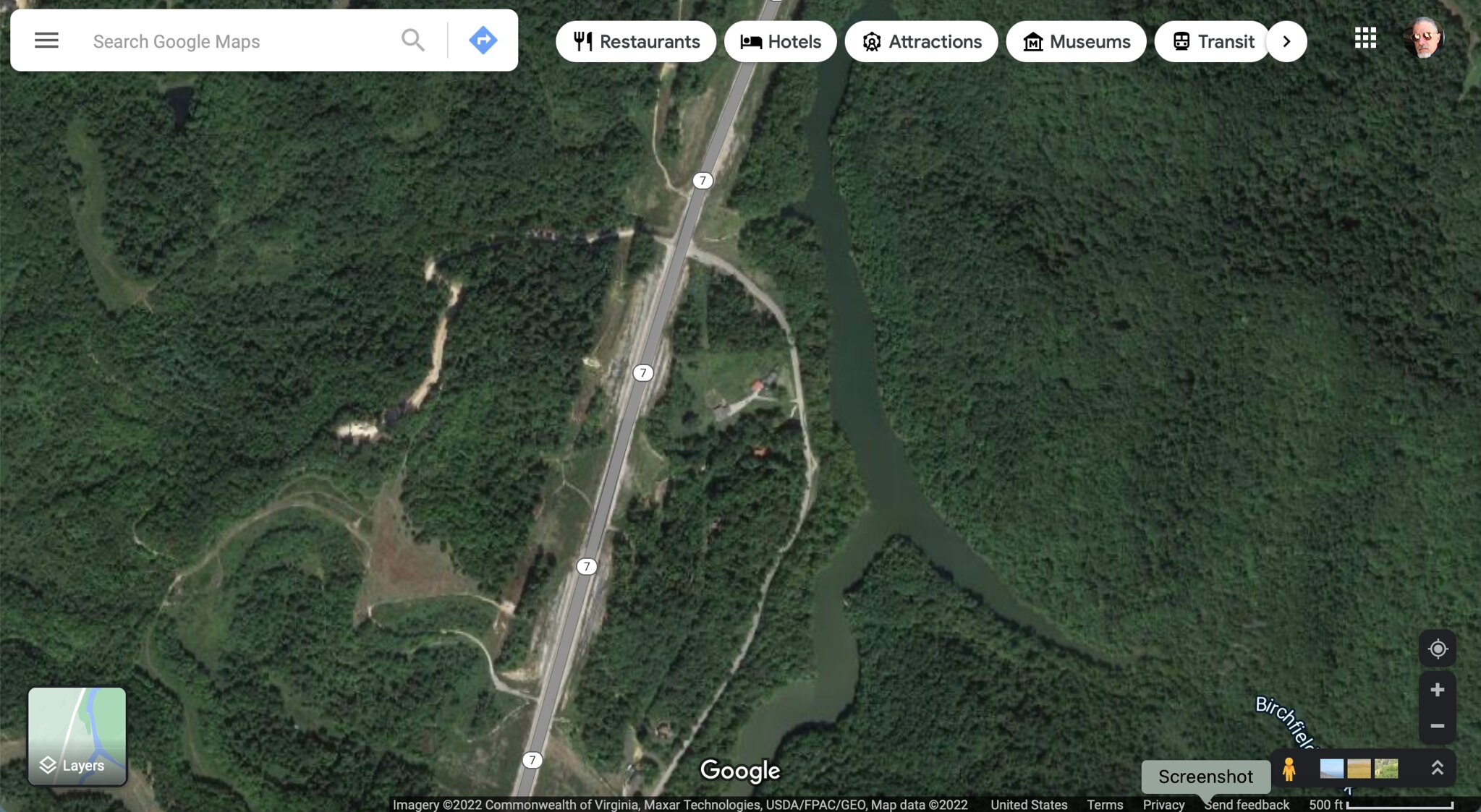This image is a detailed screenshot of a Google Maps page, presenting an aerial view of a road flanked by verdant forests and intersected by water bodies, with one identifiable street name, Burke Field, faintly visible. The top of the screenshot features the familiar Google Maps search bar on a white background. To the left of this bar are three horizontal lines, symbolizing the menu. To the right, sequentially, there is a magnifying glass icon for search, followed by a blue diamond-shaped icon with a white arrow pointing right, which usually indicates direction options. Below the search bar, five circular icons offer quick access to categories like Restaurants (signified by a fork and knife), Hotels (illustrated with a bed), Attractions, Museums (depicted by a house-like structure), and Transit (indicated by a bus). The right side of the bar shows a profile image, presumably of the user, wearing sunglasses.  

The main part of the image displays the map, showing mostly forest with a river on the right and some water areas on the left. The road running through the center is gray, with the name "Burke Field" barely legible. The bottom of the screenshot has the Google logo prominently centered. To the left, the "Layers" icon allows users to switch between different map views. On the right side, labeled in a light green box, is the word "screenshot." Adjacent to this are a small yellow figure in a square black box, additional map view options, and zoom controls (+ and -) for adjusting the focal range.